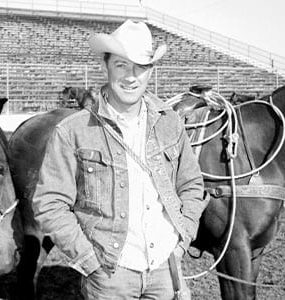In this close-up black-and-white photograph taken inside a football stadium, a cowboy stands in the center, framed from just below the crotch upward. He is wearing a white cowboy hat, a white button-up shirt, and a long-sleeved denim jacket featuring pockets above the breast. His dark blue jeans add to his classic Western attire, with both of his hands tucked into the front pockets. The cowboy has a slight smirk on his face and something resembling a rope or strap around his neck. 

To his left, part of a horse's back and a bit of its nose are visible, while to his right, another horse is seen from its midsection to the base of its neck, adorned with a saddle and a rope. Both horses are dark in color, matching the monochromatic theme of the image. The photograph’s background reveals the grandstands of the football stadium, which appear muted and empty, with large white railings and a clear blue sky above. The ground beneath them seems to be dirt, adding to the rustic ambiance, possibly indicating a rodeo event.